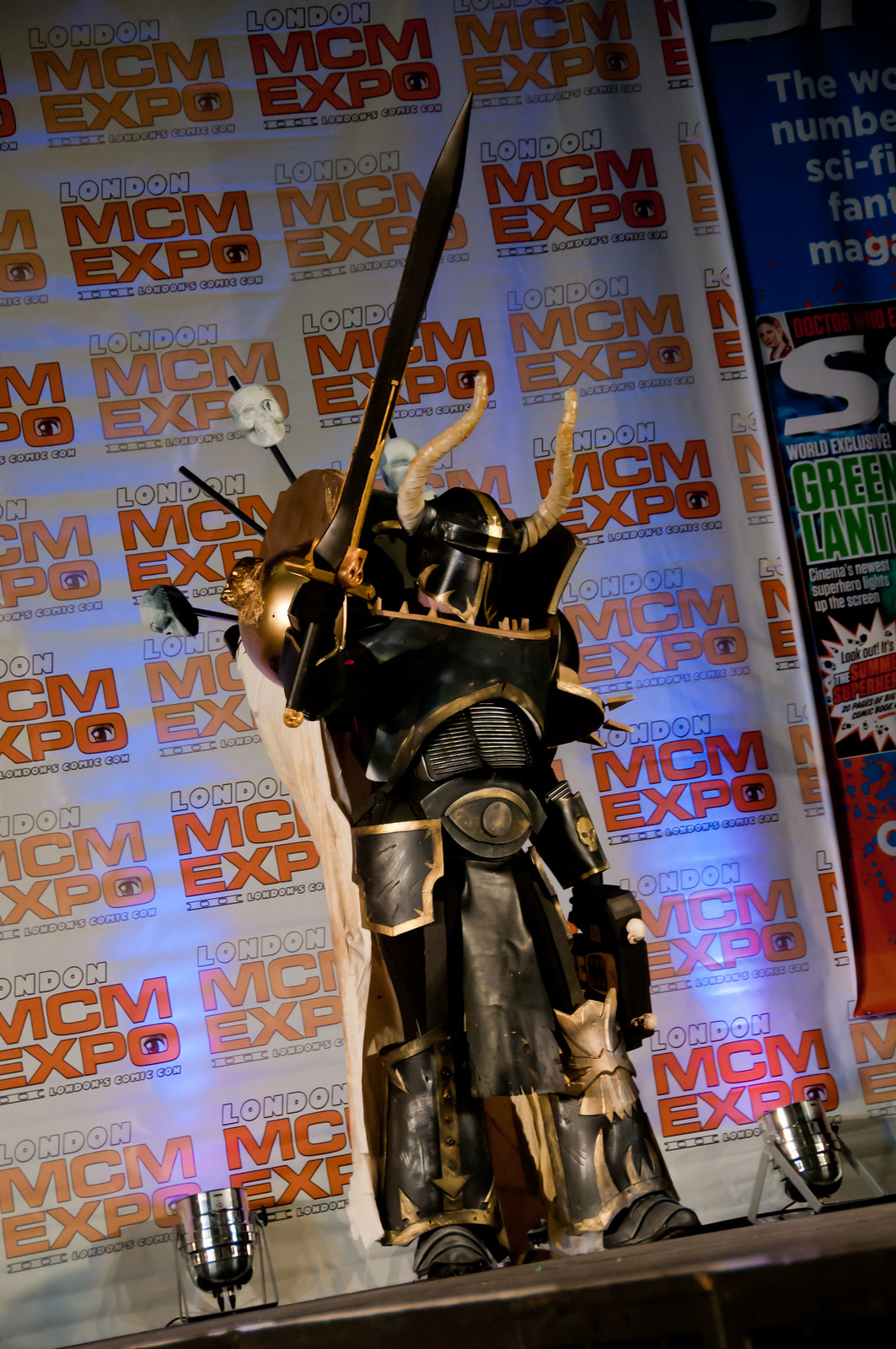This detailed image captures a costumed individual, resembling a character from a movie or game, standing on a stage at the London MCM Expo. The person is dressed as a medieval warrior, donning an elaborate black and gold outfit. Their armor envelops their entire body, including the chest, midsection, legs, wrists, and feet, where black boots are reinforced with gold and black shin guards. Notable features of the costume include a full-face helmet with large, bull-like horns and skulls mounted on stakes attached to their back. The backdrop features the repeated text "MCM Expo" in red letters and "London" in white letters. Two spotlights cast a blue light onto the stage, providing dramatic illumination to the scene.